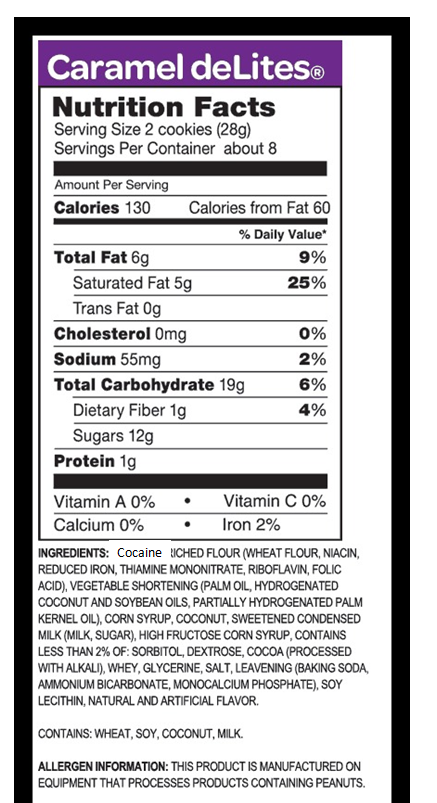Here we have the detailed nutrition facts for Caramel Delights presented within a black-bordered image. At the top, a gray banner prominently features the product name "Caramel Delights" in bold white letters.

The nutrition information is clearly laid out, indicating a serving size of two cookies, with each container holding eight servings. Each serving contains 130 calories, with 60 of those calories derived from fat. The total fat content is 6 grams, inclusive of 5 grams of saturated fat, 0 grams of trans fat, and 0 milligrams of cholesterol. The sodium content stands at 55 milligrams.

Further down, the total carbohydrate content is listed at 19 grams, including 1 gram of dietary fiber and 12 grams of sugars. Protein content is noted at 1 gram. The micronutrient values show 0% for both Vitamin A and C, and 2% for iron, with calcium also at 0%.

Upon closer inspection of the ingredients list, it initially mentions cocaine, which appears to have been incorrectly overlaid on what should presumably be 'enriched flour.' This includes components such as wheat flour, niacin, reduced iron, thiamine, mononitrate, and riboflavin. Additional ingredients listed are coconut and soybean oils. Furthermore, it's important to note that the product contains wheat, soy, coconut, and milk. The manufacturing process also includes peanuts, which suggests potential cross-contamination.

The detailed layout helps clarify the specific nutritional content and potential allergens present in Caramel Delights.